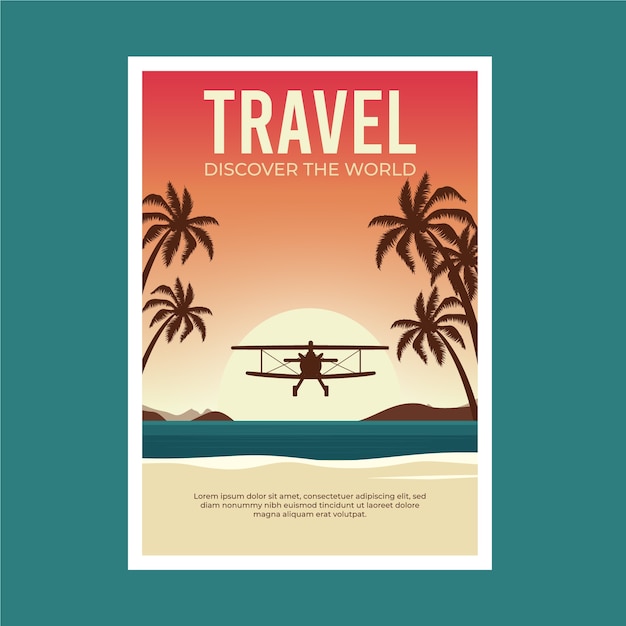This is an eye-catching travel advertisement poster with a vertical design and a green background. Inside the main aqua green square, a white-bordered brochure catches immediate attention. Dominating the center of the image is the bold title "Travel" in a vibrant gradient that transitions from red to a sunlight-inspired pale yellow. Below it, the slogan "Discover the World" is elegantly placed.

The poster's backdrop is a vivid illustration of a biplane flying towards a stunning horizon, depicting a sun either rising or setting. The sky artistically shifts from deep red to orange and culminates in a pale yellow at the sun's core. Silhouettes of palm trees flank the horizon, enhancing the tropical ambience.

Below the horizon, a body of water with a subtle bluish-green tint flows, accompanied by distant hill silhouettes. At the bottom of the image, a beach rendered in a tannish-beige hue with white-capped waves subtly grounds the design. This beach area also houses three lines of text that appear as placeholder content.

The overall composition, framed within the green square, effectively promotes the allure of travel and exploration while visually transporting the viewer to a serene, picturesque destination.